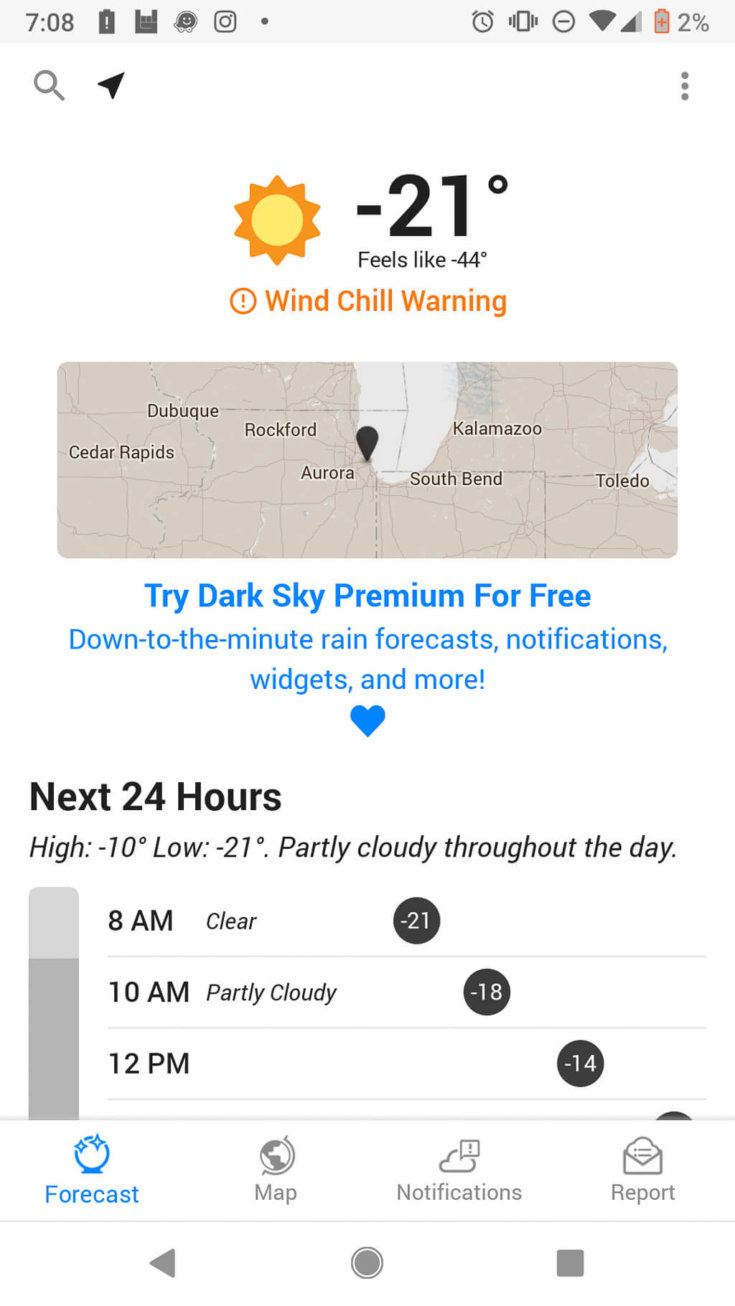The image displays the front page of a weather application on a mobile phone screen. At the top left corner, the time is shown as 7:08 p.m. An option to set an alarm is also visible. The battery icon indicates that the battery power is critically low at only 2 percent. Additionally, a search bar is positioned at the very top of the screen.

The current temperature is prominently displayed as -21°F, accompanied by a "feels like" temperature of -44°F. Despite these frigid temperatures, a bright sun icon suggests a clear and sunny day. The location is specified as Cedar Rapids, with Aurora marked to the east on the map.

A highlighted promotional banner suggests trying "Dark Sky Premium" for free, offering features like minute-by-minute rain forecasts, notification widgets, and more.

The weather forecast for the next 24 hours is detailed, stating a high of -10°F and a low of -21°F, with partly cloudy conditions expected throughout the day. Specific hourly updates are provided:
- 8 a.m.: Clear, -21°F
- 10 a.m.: Partly cloudy, -18°F
- 12 p.m.: Partly cloudy, -14°F

At the bottom of the app, the "Forecast" section is highlighted, with clickable options for "Map," "Notifications," and "Report" available for further navigation.